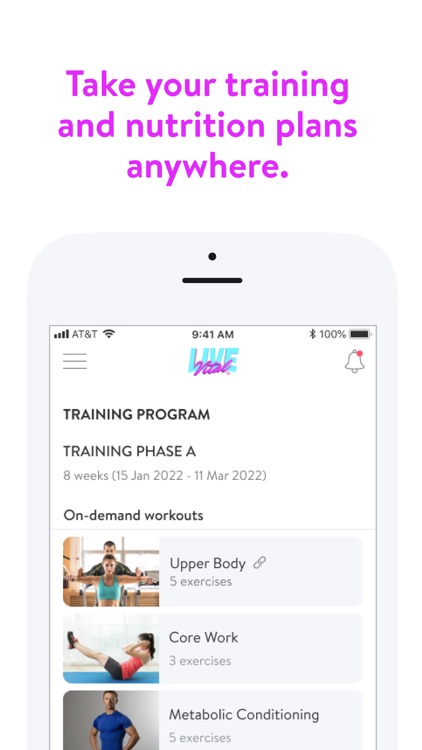The image is a screenshot captured from a mobile device, showcasing the device's faint white outline, discernible by its distinctive curved corners on the upper left and upper right sides. The screen of the mobile device itself features a sharp-cornered rectangular frame with a white background. In the upper left corner of this display, the "AT&T" logo is visible alongside the Wi-Fi icon. On the upper right, the battery icon shows a full 100% charge, and just below it, there is a notification bell with a red dot, indicating unread notifications.

The primary content on the screen is text written in black, reading as follows: "Training Program," "Training Phase A," detailing an 8-week duration from "15 January 2022 to 11 March 2022." Below this informational text, there are three smaller images, each featuring individuals engaged in various training activities, providing a visual representation that complements the training program details.